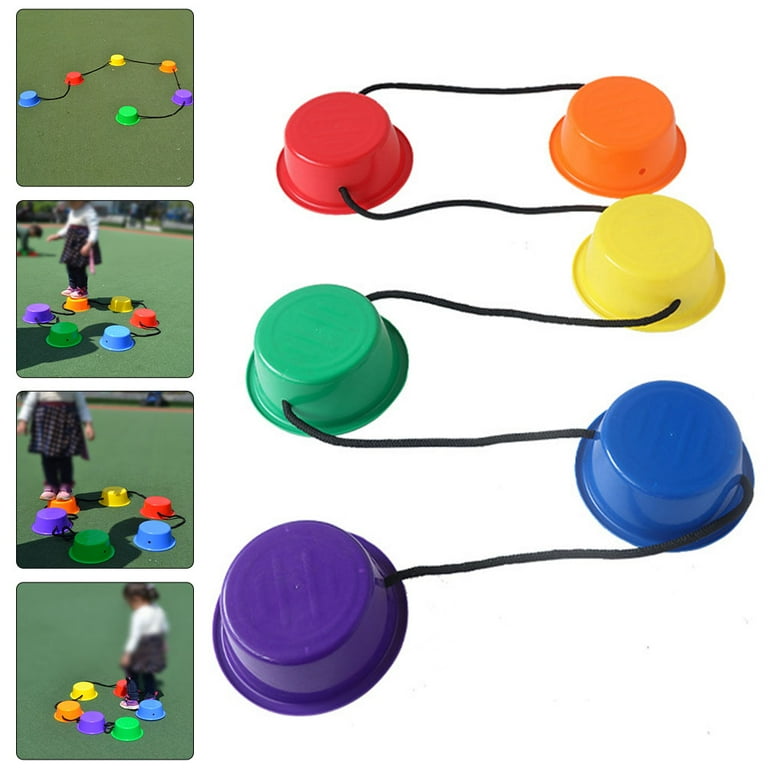The main image showcases a toy consisting of six brightly colored plastic cups—red, orange, yellow, green, blue, and purple. These cups are placed upside down in a zigzag formation, connected by a thin black cord, stretching from the back to the front of the image. The background is predominantly white. To the left, four smaller photographs are aligned vertically. The first photo displays the toy itself in a circular arrangement on grass. The second shows a little girl, blurred, standing behind the circle of cups. In the third image, the girl, whose feet rest on an orange cup, appears to navigate a path on top of the cups. The final photo captures her from behind, standing between two of the cups. The sequence of images suggests that the toy's objective is for children to balance and move from cup to cup without touching the ground.